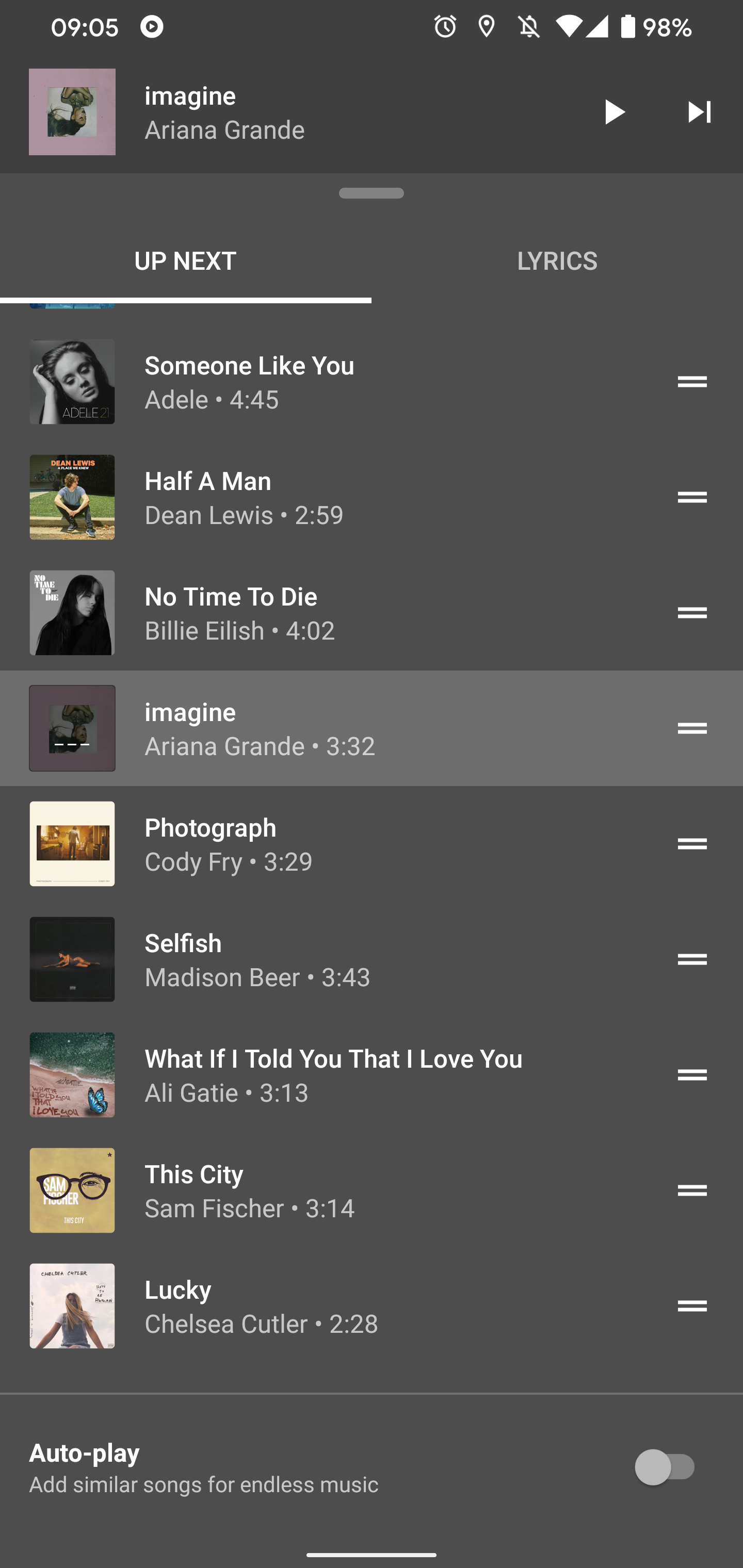The image is a screenshot from a smartphone set in dark mode. In the top left corner, the time is displayed as 9:05, followed by a series of status icons: a black mark inside a white circle, a timer icon, a location on icon, a sound off icon, a Wi-Fi icon, a fully charged battery icon, a camera icon, and the battery percentage which is at 98%.

Below the status bar, there's an album cover image labeled "Imagine" by Ariana Grande. Underneath that, on the left side, it says "Up Next," with "Lyrics" displayed horizontally across from it. 

The list of upcoming songs includes:

1. "Someone Like You" by Adele (4:45) accompanied by her picture.
2. "Half a Man" by Dean Lewis (2:59) with his picture.
3. "No Time to Die" by Billie Eilish (4:02) along with her picture.
4. "Imagine" by Ariana Grande (3:32) with what seems to be her image, although it's not very clear.
5. "Photograph" by Cody Fry (3:29) alongside the album cover.
6. "Selfish" by Madison Beer (3:43) paired with an album cover image.
7. "What If I Told You That I Love You" by Ali Gatie (3:13) next to an album cover.
8. "The City" by Sam Fisher (3:14) with an image of a pair of glasses.
9. "Lucky" by Chelsea Cutler (2:28) with her picture.

At the bottom, there is an "Autoplay" toggle accompanied by a description: "add similar songs for endless music."